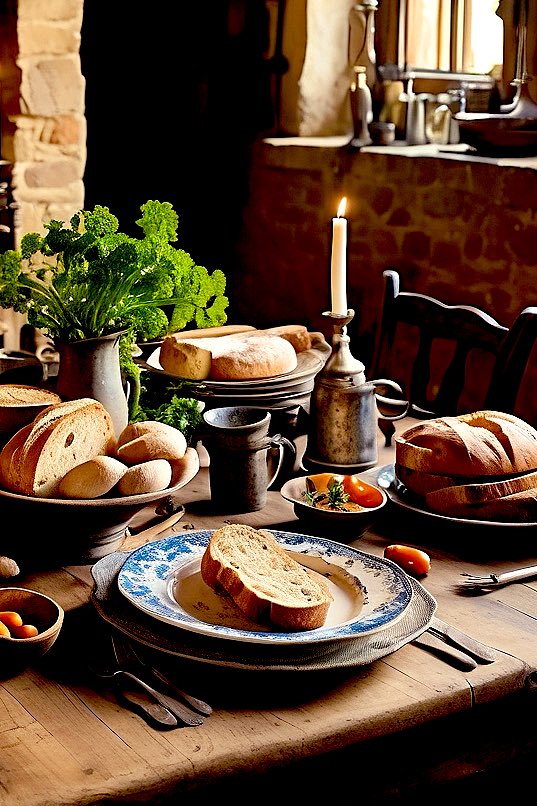The color photograph showcases a beautifully set rustic kitchen scene within a stone-walled building, bathed in natural sunlight filtering through a window. At the forefront, a dark wooden table is meticulously arranged with an array of different breads. On the left, a plant in a ceramic vase adds a touch of greenery, while beside it, a stack of plates holds various loaves and slices of bread. Another plate adorned with a blue and white floral pattern contains soup and a slice of bread. 

In addition, there's a metal candle holder with a lit taper candle and a matching tarnished tin cup, evoking a historical ambiance. Scattered across the table are multiple plates and bowls: one containing cherry tomatoes or small round vegetables, another with a medley of bread types – some whole, some sliced. A notable plate with a blue china pattern highlights the table's assortment. Silverware is neatly placed next to the plates, completing the setting. Behind the table, the scene is framed by a stone pillar and a stone countertop with a collection of containers, enhancing the rustic aesthetic. The overall arrangement gives the impression of a recreated old kitchen, steeped in charm and history.